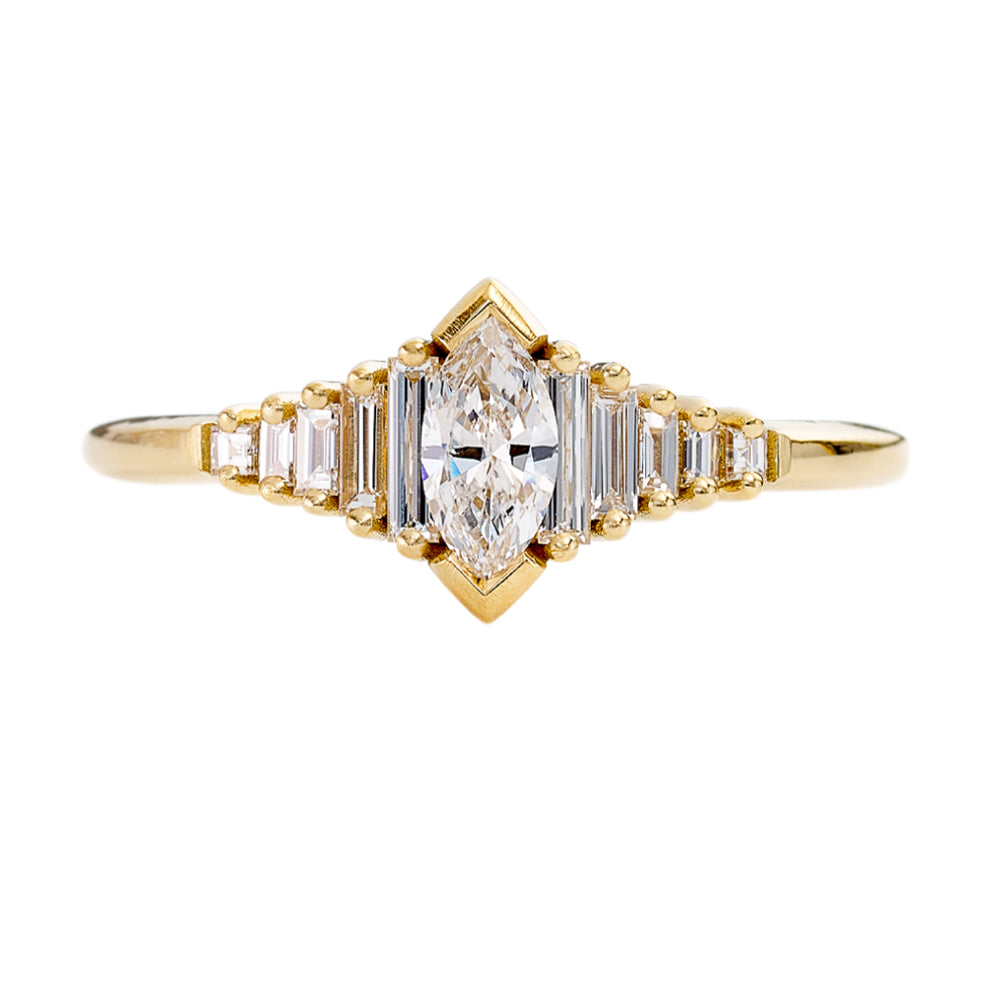The image features an elegant and seemingly expensive ring set against a plain white background. The ring's band, approximately 4 inches wide from left to right, is crafted from narrow gold that subtly transitions to a silver tone as it curves around the back. Central to the ring's design is a striking leaf-shaped diamond or possibly a similarly reflective cubic zirconia, slightly under an inch in length but expanding closer to an inch when considering the surrounding gold bands. This prominent stone reflects hints of black and blue, adding to its allure.

Flanking the central jewel are a series of smaller rectangular cubic zirconias, which gradually increase in size towards the center. The top and bottom of these stones are adorned with delicate gold spheres. The overall ring composition includes 11 diamonds or diamond-like stones, showcasing a masterful step-like arrangement around the centerpiece. These stones shimmer across a spectrum of colors depending on the lighting, further enhancing the ring's luxurious appearance. The intricate design is accentuated by a triangular pattern of gold ornamentation running vertically along the central stone, adding a distinctive and sharp geometric elegance to the piece.